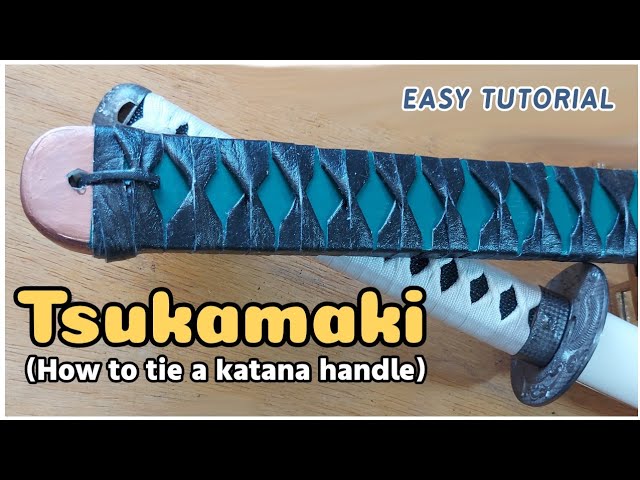This image is a thumbnail for a YouTube video tutorial detailing "How to Tie a Katana Handle." In the upper right corner, there is blue text with a white outline that reads "Easy Tutorial." Prominently in the bottom left corner, larger bright yellow text states "Tsukamaki," and underneath, white text in parentheses elaborates with "how to tie a katana handle." The scene features a katana with a white blade and handle resting on a light brown wooden table. The katana's casing, exhibiting a black pattern with blue underneath, takes prominent focus. The handle appears to be wrapped with a shiny blue material, possibly leather or vinyl. The entire image has thick black borders at the top and bottom, suggesting it was likely screenshotted from a video platform, confirming typical YouTube dimensions.